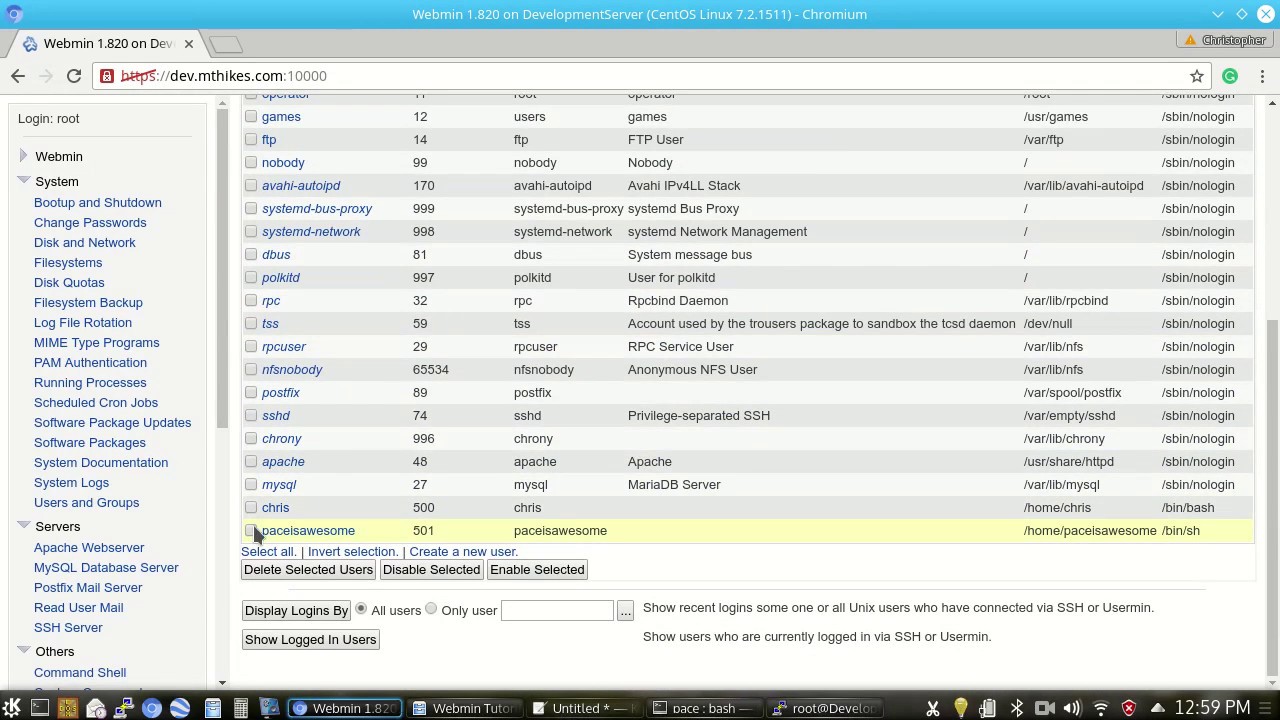Here is a cleaned-up and detailed caption for the image you described:

---

This image showcases a user's desktop displaying the Webmin application, version 1.8.20, accessed on a development server. The browser's URL bar, showing "https://dev.mthikes.com:10000", has the HTTPS crossed out with a red line, indicating a potential issue with the security certificate. Only one browser tab is open.

The Webmin interface itself reveals a detailed table spanning six visible columns. Although the column headers are not in view, the first column comprises a variety of manually assigned variable names. Adjacent columns contain numerical values and various labels. Notably, the last column predominantly features entries like "/sbin/nologin", "/bin/dash", and "/bin/sh", suggesting user account configurations, possibly shell access details.

Along the left side of the Webmin interface, there's an extensive list of hyperlinks, each leading to different sections or configurations within the Webmin setup, hinting at the administrative capabilities and breadth of control provided by the application.

---

I hope this provides a clear, detailed description of the image.